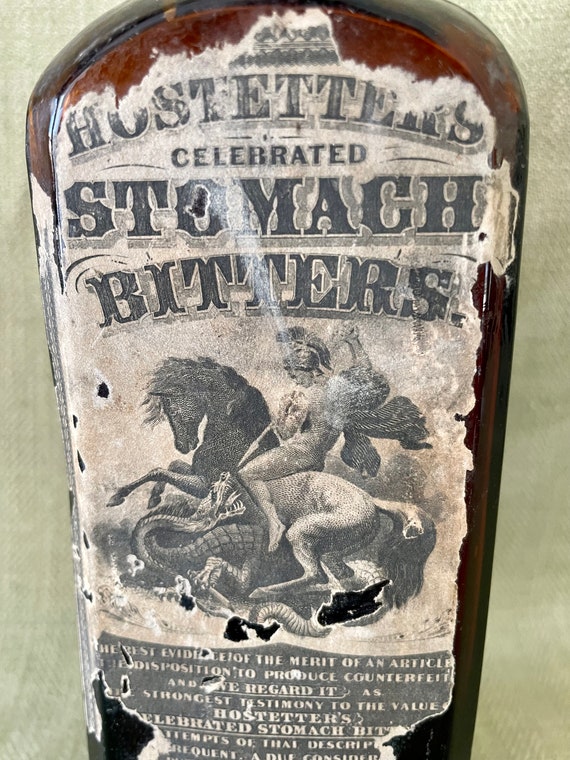The image features an old, brown bottle displayed against a greenish-gray background. The bottle has a very worn and almost torn label that is predominantly in black and white. The label indicates that the bottle contains "Haas Stillers, celebrated stomach bitters." The focal point of the label is an intricate etching of a dramatic scene: a helmeted, naked man on a rearing horse is attempting to spear a snake that threatens them. The label is highly faded and contains text that is difficult to read due to numerous small holes. However, part of the text reads, "strongest testimony to the value, Haas Stillers, celebrated stomach bitters." The bottle itself is centered in the frame, with its colors blending with the surrounding hues of pale greens, blacks, grays, and browns, contributing to the antique aesthetic captured in the image.